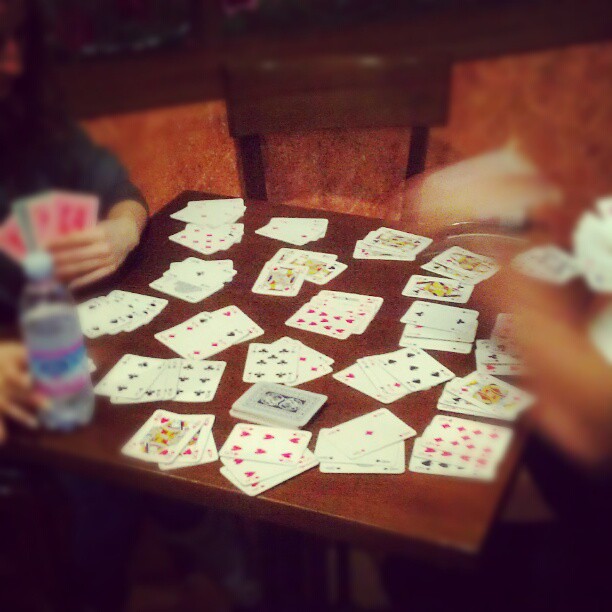In this photograph, we see a lively scene of two individuals engaging in a card game at a small poker table. On the left-hand side, there is a man holding up cards in his left hand. He has three cards with red backs and one card with a gray or blue back. He is also holding a bottle of water in his right hand, and he is wearing a dark bluish t-shirt. 

On the right-hand side, there is another person, although this individual is completely out of focus, possibly due to motion blur, making it difficult to discern their features. 

The table itself is a rich cherry wood, and it is covered with several neatly arranged sets of cards. These sets each consist of three cards, such as three queens, three jacks, three fours, three fives, etc., totaling around 15 to 18 different sets. At the bottom center of the table, there is a somewhat depleted deck with approximately 20 cards remaining, indicating that they have been playing for quite some time.

The backdrop features a dark reddish maroon wall, adding to the warm ambiance of the room. The scattered arrangement of cards on the table further suggests that the game has been ongoing for several hours and may be approaching its conclusion as the deck continues to dwindle.